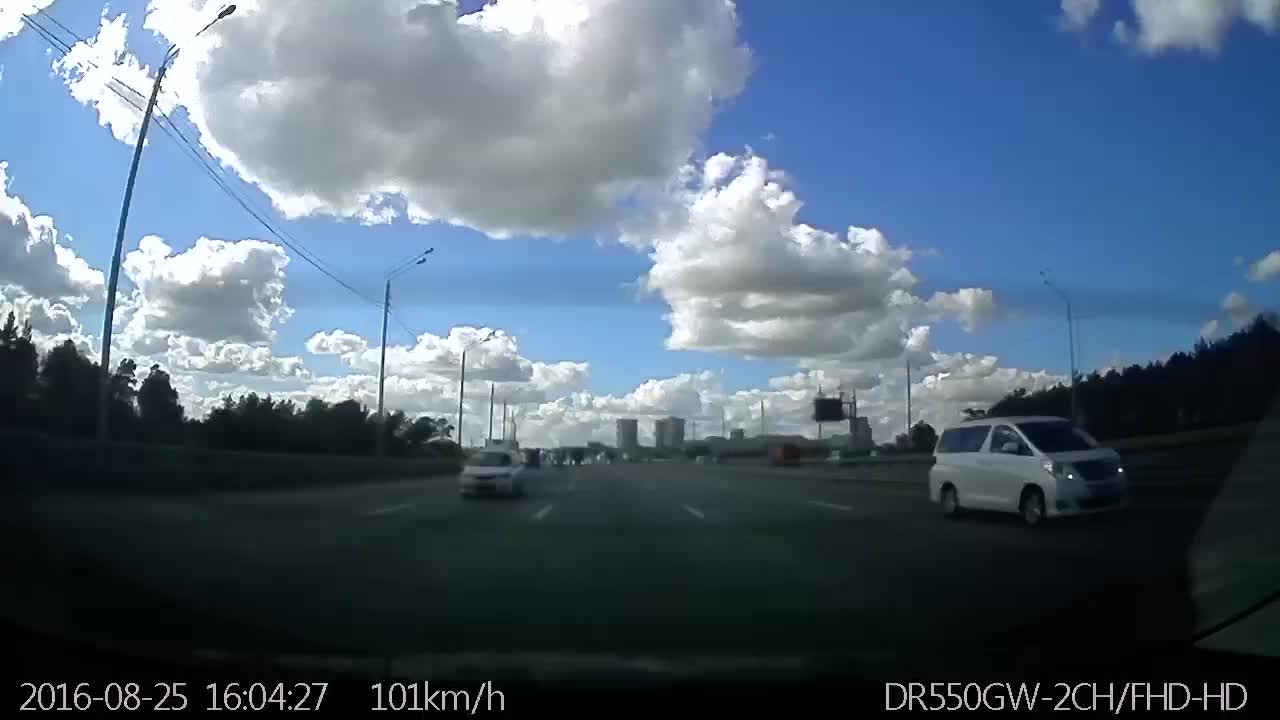A large rectangular image captured by a rear-facing camera on a vehicle presents a detailed scene of a five-lane freeway. The bottom edge of the image is overlaid with camera information, featuring the date and time on the bottom left, the vehicle's speed in miles per hour in the center left, and additional camera details on the right. The image has a slight fisheye effect likely caused by the camera lens, providing a rounded view of the surroundings. 

In the background, two white vehicles are visible: a white minivan traveling in the far right lane and a small white sedan positioned to the left of the vehicle with the camera. The sky above is a clear blue, adorned with large white clouds. In the distant background, a cityscape of buildings is visible, adding depth to the scene. The far left side of the freeway is bordered by trees and power lines, adding a touch of greenery to the urban environment.